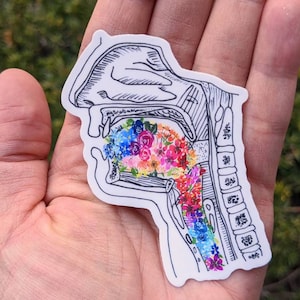A close-up photograph captures a Caucasian person's left hand, palm up, against a background of green grass. Positioned in the center of the palm is a white sticker featuring a detailed black-and-white medical diagram of a human head and neck in profile, illustrating the nasal passages, mouth, throat, and spinal column. The mouth and throat areas of the diagram are brightly adorned with colorful flowers in shades of blue, pink, orange, and yellow, giving a child-like, whimsical contrast to the clinical sketch. The diagram, reminiscent of an x-ray, distinctly shows the nostrils, an open mouth, and segmented spine, though cut off right below the neck.